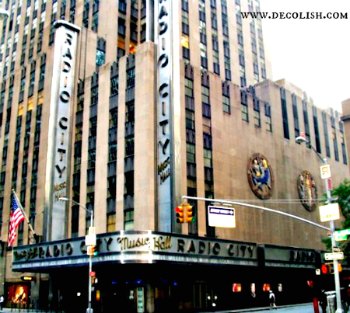The image depicts an urban scene featuring the iconic Radio City Music Hall in New York City. The centerpiece is a tall, tan-colored building with black windows, extending beyond the frame. Prominently displayed on the building are two vertical signs that span several stories, both emblazoned with "Radio City Music Hall" in bold text. One sign is situated to the left and stretches across seven stories, while the other is about four windows away, similarly labeled. At the center where the building’s corner bends, the marquee wraps around, showcasing "Music Hall" in elegant gold script alongside "Radio City" on both sides, accentuated by a blue line and a gray strip. Higher up, the facade features round decorative elements. An American flag flutters from a flagpole on the left side of the building. Adjacent to this, a streetlight and support beam are visible, along with several traffic signs. The street level beneath the marquee appears dark, in contrast to the bright daylight illuminating the rest of the scene. In the background, other tall buildings and urban features, like trees and sidewalks, underscore the bustling city environment.